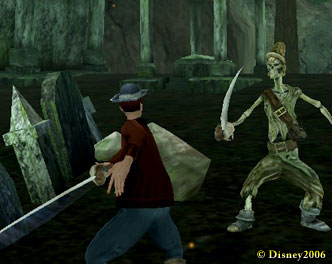The image depicts a cartoon scene, possibly from a video game or animated show, featuring a dramatic encounter between two characters. A skeleton dressed in raggedy clothing, with torn trousers and a worn jacket, stands armed with a sword. Opposing the skeleton is a man with short brown hair, fair skin, and his back towards the viewer. He is attired in a brown shirt and blue pants, topped with a gray hat. The man appears to be fleeing, clutching a large sack. This tense standoff unfolds on a dark surface, likely within a graveyard or similar eerie setting, hinted at by the presence of fencing or tombstones scattered around. Adding a layer of authenticity to the image, the bottom right corner features a faint yellow Disney logo, with a copyright mark dated 2006.